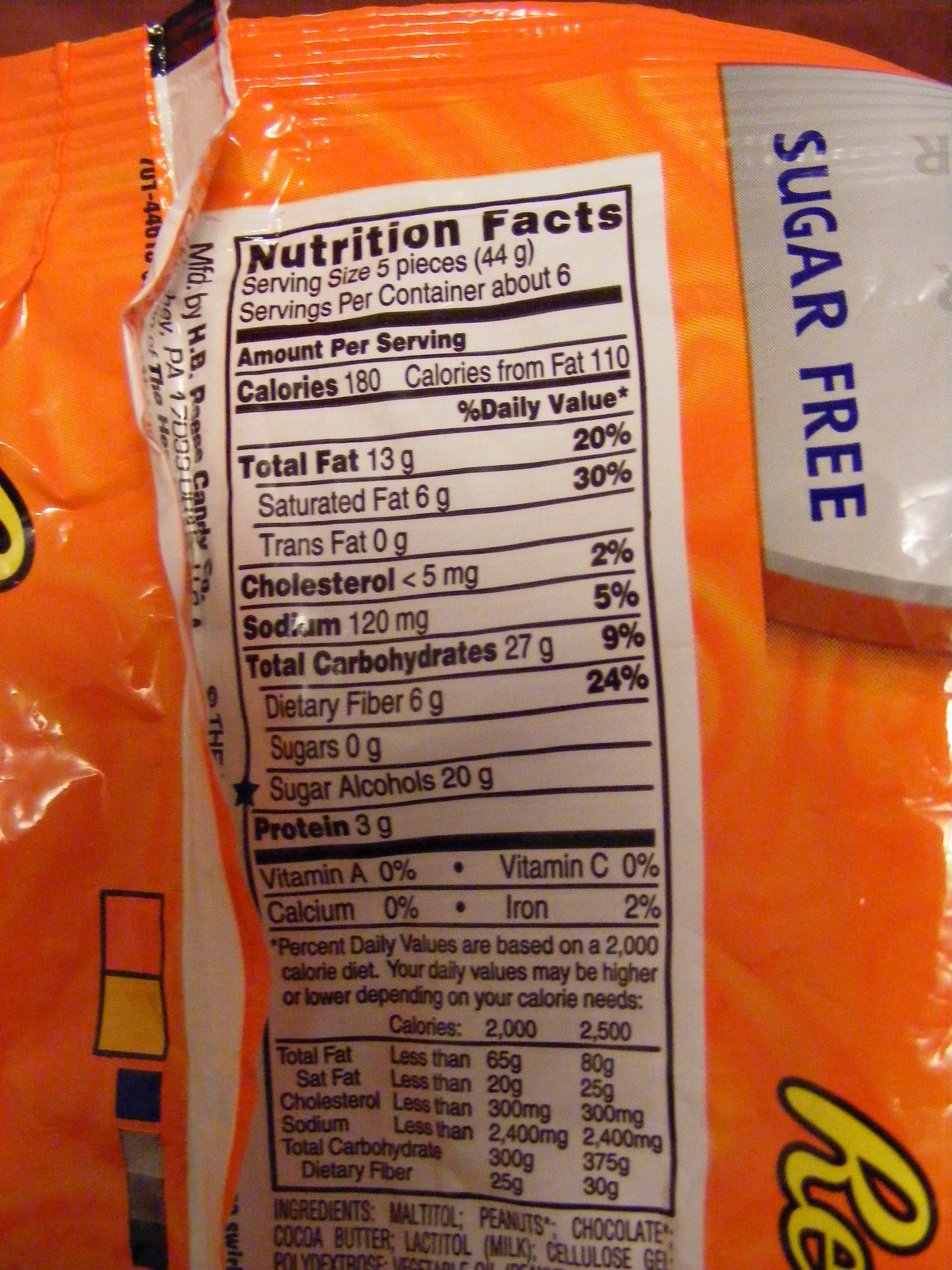Here is a detailed and cleaned-up caption for the image:

"A vibrant orange bag of Sugar-Free Reese's is prominently displayed. The familiar ‘RE’ and signature Reese's branding are visible on the packaging, along with a clear label indicating that these treats are sugar-free. The nutrition facts on the back of the package reveal important details: the serving size is five pieces with about six servings per container. Each serving provides 180 calories, 110 of which are from fat. The total fat content is 13 grams, making up 20% of the daily value, with 6 grams of saturated fat (30% DV) and no trans fat. The cholesterol count is 5 milligrams (2% DV), and the sodium content is 120 milligrams (5% DV). There are 27 grams of total carbohydrates (9% DV), with 6 grams of dietary fiber (24% DV) and 20 grams of sugar alcohols. The protein content is 3 grams per serving. Notably, the amounts of Vitamin A, Vitamin C, and calcium are 0% of the daily value, while iron contributes 2%."